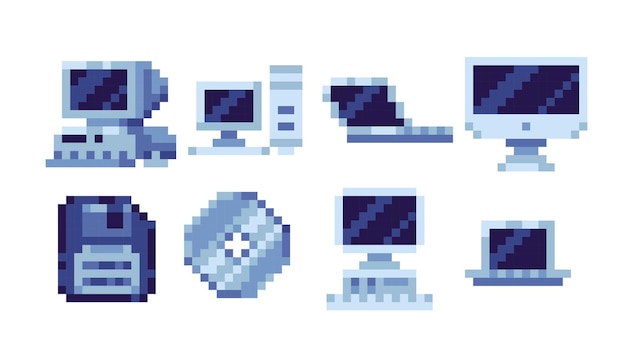This image features eight pixelated illustrations of various computers and peripherals, organized in two rows of four against a backdrop of blue and dark blue hues. Starting from the left in the top row, the first illustration depicts an old-fashioned CRT monitor resting atop a horizontal base, followed by a classic desktop setup with a monitor standing beside its tower. Next to it, there is an image of what appears to be a laptop, and at the top right, a standalone monitor with a multi-layered stand is displayed. Moving to the bottom row, the first illustration on the left is of a floppy disk, followed by what looks like an image of a CD case or badge formation with a cross in the center. The seventh illustration features a monitor placed on a horizontal desktop, and finally, the last image in the bottom right is a short monitor. The pixelation gives each component a retro, blocky appearance reminiscent of early digital graphics.